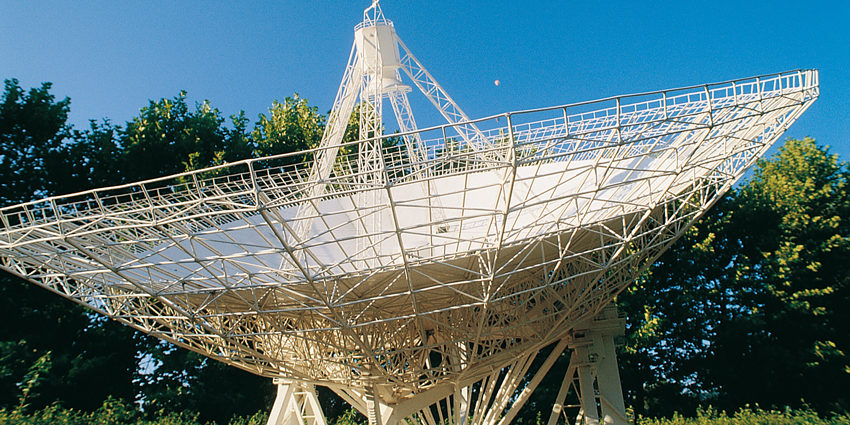This outdoor photograph, taken during the daytime in a landscape orientation, captures a large beige-white satellite dish standing prominently in an open field. The satellite dish, which is tilted slightly to the left and pointing towards the upper right corner, dominates the bottom two-thirds of the image. The dish itself features a wire frame with a solid interior and is supported by several vertical pillars—at least three forming the base and four metal grid columns converging towards a central peak at the top. Surrounding the base is a lush green field, dotted with rows of hedges and bushes, which allow glimpses of the deep blue sky behind. Two small, hot air balloon-like dots are visible near the upper right of the satellite dish. The panoramic view culminates in a stunning expanse of blue sky, stretching above the greenery.